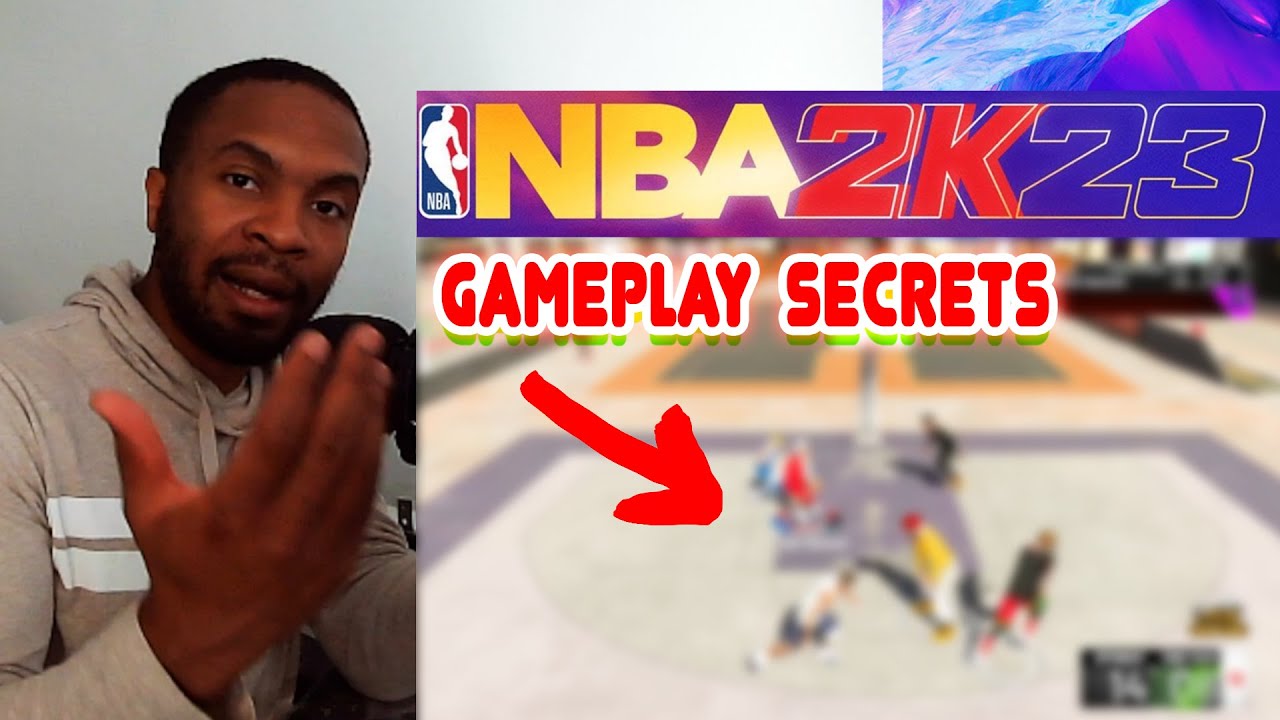In this image, an African-American man is positioned towards the left side, actively explaining or describing something. On the right side of the image, there are gameplay secrets from the video game NBA 2K23 being showcased. A red arrow is prominently pointing towards the center, directing attention to the characters involved in the gameplay. The scene is vibrantly colored with shades of yellow, red, blue, purple, brown, and white, creating a visually engaging composition.